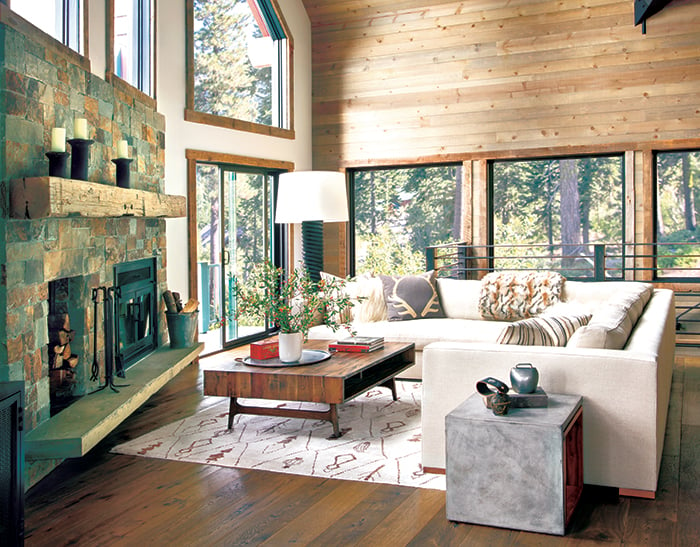This spacious and rustic living room boasts large square glass windows that bring the lush, green forest surroundings inside, creating a serene and isolated ambiance. The focal point of the room is its unique double fireplace set into a large, textured stone wall to the left, flanked by twin hearths— an uncommon and eye-catching feature. 

The back wall is adorned with natural wood planks, reinforcing the rustic aesthetic, with floor-level windows providing an immersive view of the trees outside. The white couches, arranged in an L-shape, are adorned with assorted pillows, including a gray one and a striking black-and-white striped pillow. Below the sofa lies a white rug with intricate designs.

At the center of the room, a rectangular brown wooden coffee table holds a white potted plant and scattered books, adding to the cozy, lived-in feel. Above the fireplace’s wooden mantel, a selection of white candles with dark accents creates a charming contrast. The high, white ceiling and walls amplify the room's brightness, further enhanced by additional windows and a sliding door on the left, which invites more natural light and connects the indoor space seamlessly with the outdoors.